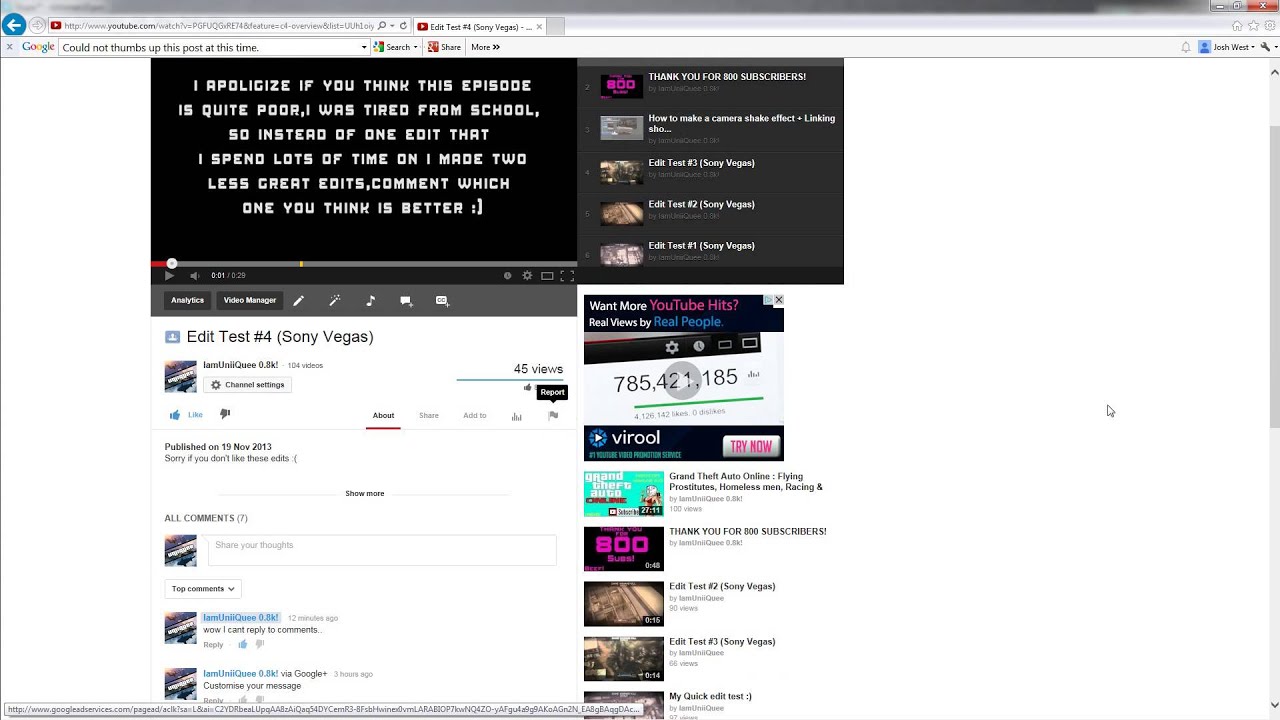The image depicts a screenshot from a YouTube video page. At the top, the URL bar displays "YouTube.com/watch" followed by a string of letters and numbers, indicating a specific video. The title of the editing project, "Edit Test Number Four, Sony Vegas," is visible, suggesting that the video was created using Sony Vegas software. 

There is a message box from the Google app stating "Could not thumbs up this post at this time," implying an issue with liking the content. The video in question is 29 seconds long, with only one second played, as indicated by a small red progress line at the beginning, while the remainder of the progress bar is gray.

Within the video post, there is a text overlay in bold, all-caps, block letters: "I APOLOGIZE IF YOU THINK THIS EPISODE IS QUITE POOR, I WAS TIRED FROM SCHOOL, SO INSTEAD OF ONE EDIT THAT I SPEND LOTS OF TIME ON, I MADE TWO LESS GREAT EDITS. COMMENT WHICH ONE YOU THINK IS BETTER :)." Beneath the post, there are various clickable areas where users can view and leave comments.